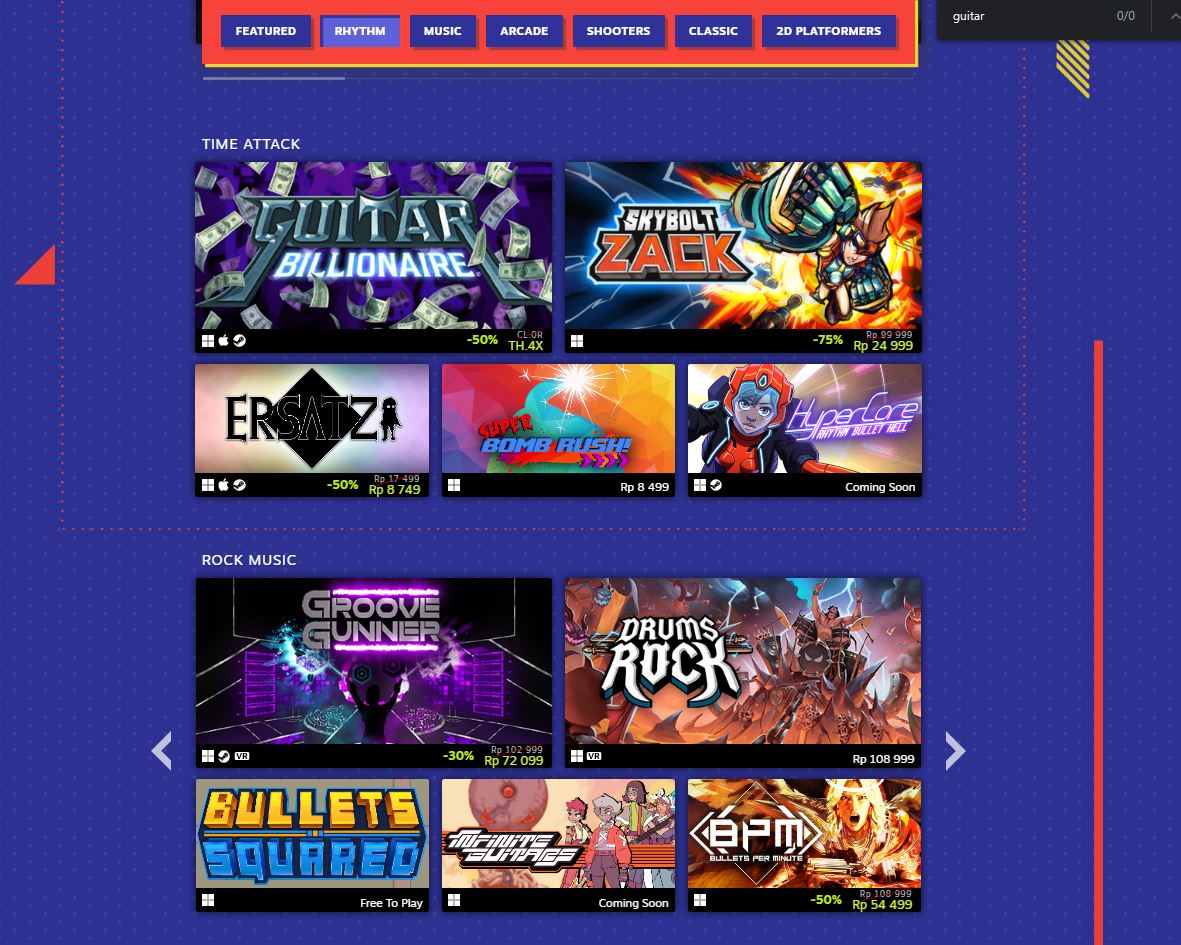The image features a square layout with a royal blue background interspersed with tiny, faint white dots. At the top center of the image, a horizontal red banner stretches partway across the width. This banner houses a navigation menu with blue buttons bearing white text, labeled "Featured", "Rhythm", "Music", "Arcade", "Shooters", "Classic", and "2D Platformers". The "Rhythm" button is highlighted, indicating it has been selected. 

To the far right of this banner is a short black search bar containing the word "Guitar" in white text. Directly below the banner, the white text "Time Attack" is prominently displayed, followed by a grid of game titles with corresponding images. The games listed under this category are "Guitar Billionaire", "Skybolt Zack", "Ersats", "Super Bomb Rush", and "Hypercore".

A short space separates the "Time Attack" category from the next, labeled "Rock Music" in white text. The games displayed under this section include "Groove Gunner", "Drums Rock", "Bullets Squared", "Infinite Guitars", and "BPM: Bullets Per Minute". 

To the right of the image, a slender vertical red line extends from the "Time Attack" heading to the bottom edge. Adjacent to the "Rock Music" game titles, there are forward and backward navigation buttons to scroll through additional game options.